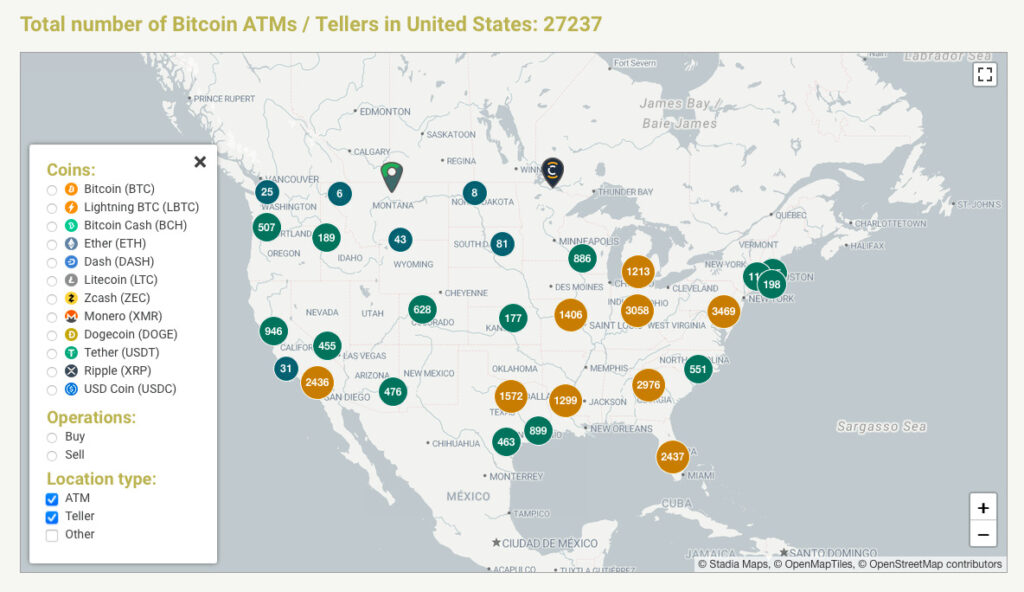This detailed map of the United States, along with portions of Canada and Mexico, showcases the distribution of Bitcoin ATMs across various regions. The map highlights a total of 27,237 Bitcoin ATMs/tellers in the United States. An extensive key on the left side explains the data points: 

- **Coins Supported:** Bitcoin (BTC), Lightning Bitcoin (LBTC), Bitcoin Cash (BCH), Ether (ETH), Dash (DASH), Litecoin (LTC), Zcash (ZEC), Monero (XMR), Dogecoin (DOGE), Tether (USDT), Ripple (XRP), USDCoin (USDC). 
- **Operations Available:** Buy, Sell.
- **Location Types:** ATM teller and other, with 'ATM teller' selected.

Highlighted regions on the map include:

- **Miami, Florida:** 2,437 ATMs.
- **Ohio:** 3,058 ATMs.
- **Michigan:** 1,213 ATMs.
- **Kansas:** 177 ATMs.
- **San Diego, California:** 2,436 ATMs.

This comprehensive depiction provides a clear visualization of Bitcoin ATM accessibility, emphasizing areas with high concentrations of these cryptocurrency facilities.